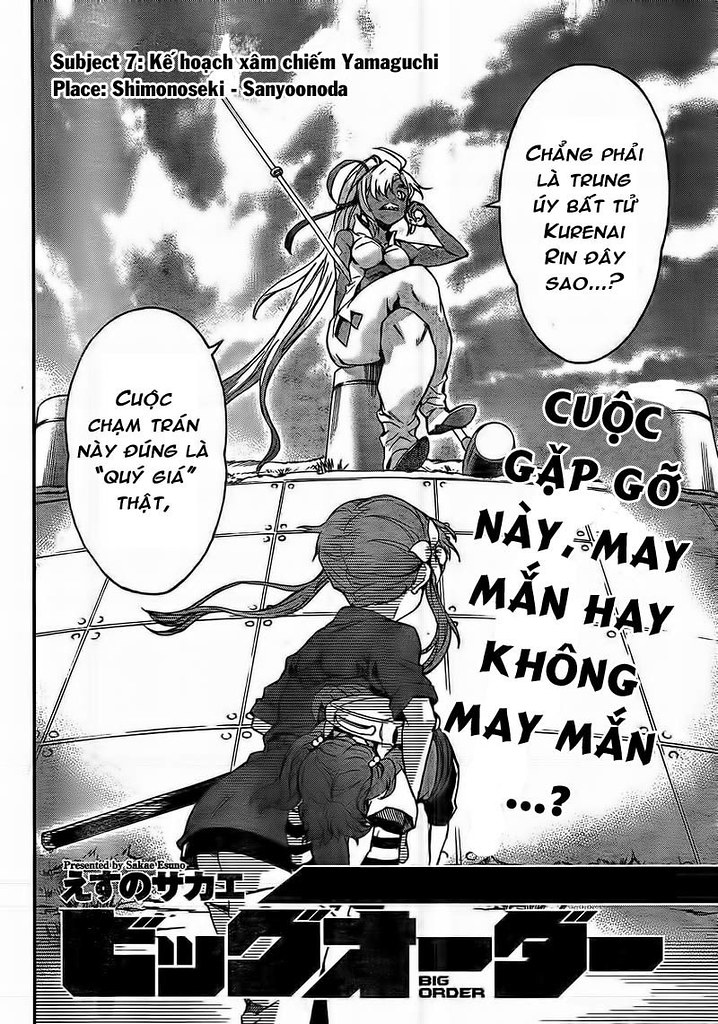The black and white image appears to be a page from a comic book, possibly the front page of an issue or a part of a magazine featuring comical or anime-style drawings. The heading on the top left reads "Subject 7" alongside some foreign characters which seem to be in an Asian language, potentially Thai or Japanese. The scene displays multiple characters, one facing forward and another shown from the back, distinguished by their contrasting features; the first with dark skin and blonde hair, and the second with light skin and dark hair. A centrally positioned animated image of a woman with long hair clad in a white bra and pants captures attention, accompanied by word bubbles on her right and left, filled with text in an unreadable Asian script. Additional foreign text is present at the bottom right and across the lower section of the page, with the term "Big Order" appearing prominently.